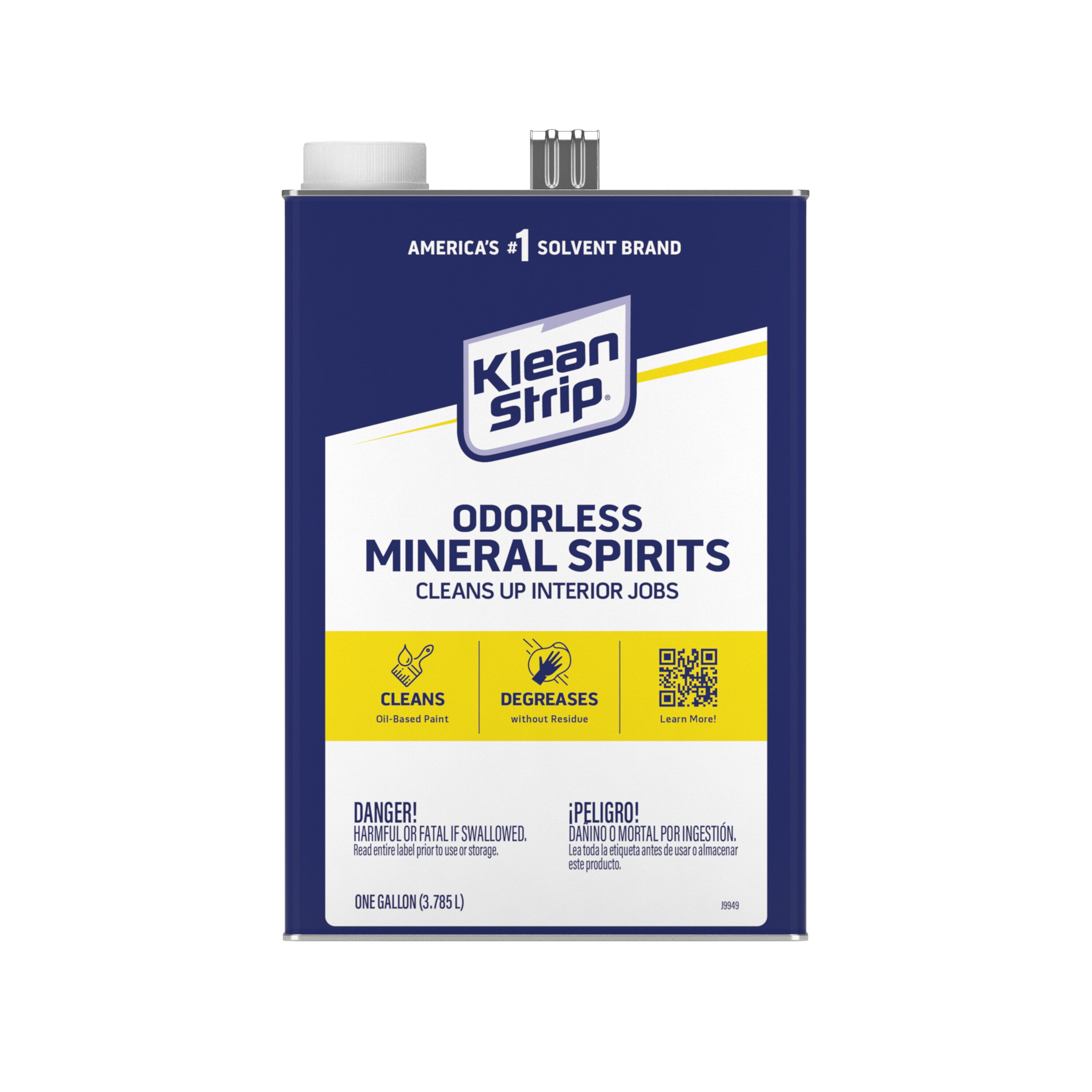The image shows a metal canister with a dark blue background, prominently featuring the branding and details of an America's number one solvent brand product called Clean Strip. The canister is topped with a white plastic screw-on cap. Across the top of the canister, in white text, it boldly states "America's number one solvent brand." Below this proclamation is a logo with a blue border, white background, and a yellow diagonal stripe running through it, stating "Klean-Strip." Directly beneath the logo, it reads "odorless mineral spirits" in blue text on a white background, with additional text "cleans up interior jobs." There is then a yellow stripe highlighting specific uses: a small paintbrush icon with the text "cleans oil-based paint," and a hand with a rag icon indicating it "degreases without residue." A QR code to "learn more" is also present. Towards the bottom, various warning labels are displayed, stressing the product is "dangerous and harmful or fatal if swallowed," with this warning repeated in Spanish to the right. In the bottom left corner, the volume is marked as "one gallon (3.785 liters)."